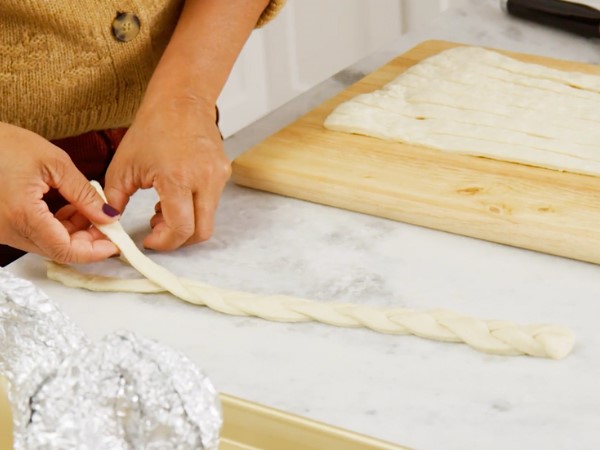In this detailed indoor kitchen scene, a woman is demonstrating how to make bread. Only her waist and hands are visible, as she twists or braids the dough on a white and gray marble countertop dusted with flour. She is dressed in burgundy pants and a tan knitted sweater adorned with tortoiseshell buttons, and her fingernails are painted a dark burgundy or dark brown shade. On the countertop, a large light wooden cutting board is placed, holding flattened dough that has been cut into strips. Additional strips of dough lie on the board, awaiting braiding. In the bottom left corner of the image, there is some crumpled aluminum foil. In the background, a white door is visible, contributing to the cozy kitchen setting.